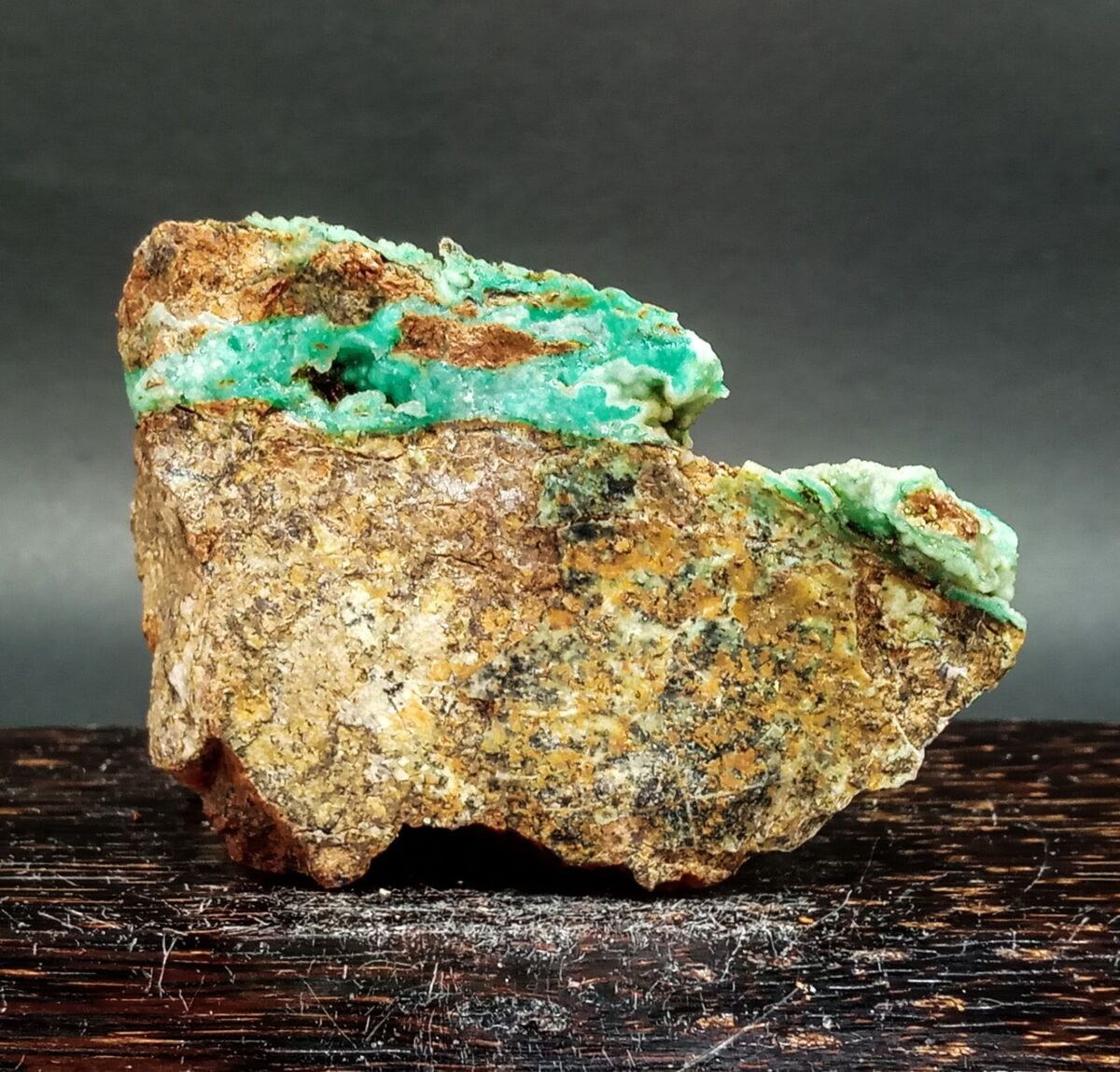The image depicts an irregularly shaped rock resembling a flipped stomach, resting on a scratched and chipped black wooden surface with a gray background. The rock's body primarily exhibits a color similar to cooked chicken, interspersed with small dots that give it a seasoned appearance. The upper portion of the rock features a striking gem-like section, transitioning from a light blue to a greenish hue, reminiscent of jade. This colorful element sprawls from the top left to right, weaving through the rock's natural grooves. Additionally, the rock displays a variety of hues, including light tan, gray, almost white, and sections of brown, particularly noticeable on the bottom left. This intricate blend of colors and textures creates a unique, visually engaging crystal-like formation.